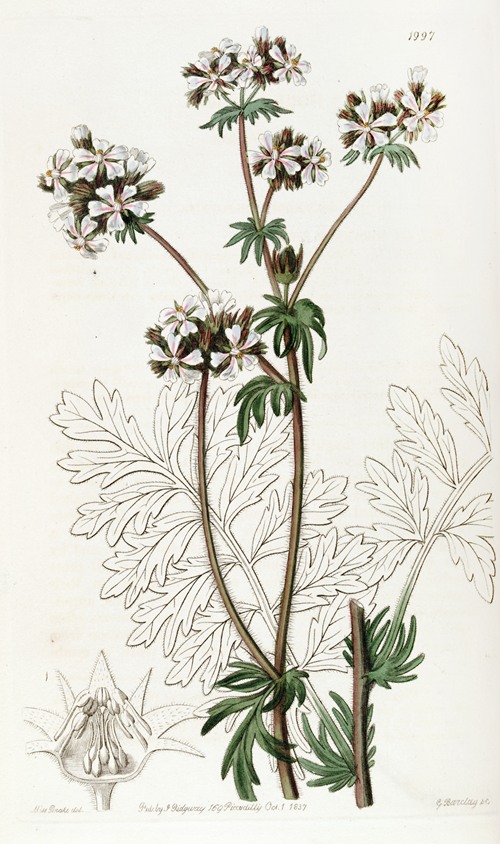The image is a tall, rectangular illustration dominated by a detailed drawing of a skinny, tall plant. The background is a pale white or light beige, contrasting with the more vibrant elements of the plant. In the top right corner, small text indicates the year "1997". The plant features brownish branches and green, palmate leaves with a pointy shape. Some of the branches are unfinished sketches in black, adding a dynamic preliminary touch to the artwork. Clusters of white flowers, each with five petals, are scattered towards the top of the plant, standing out against the pale background. Additionally, white leaves emerge from some branches, which are also depicted in white. In the bottom left of the image, a close-up illustration of a flower is mostly white with some scribble-like details. Tiny, barely visible text is at the bottom of the image, enhancing the intricate and detailed style of this floral illustration.